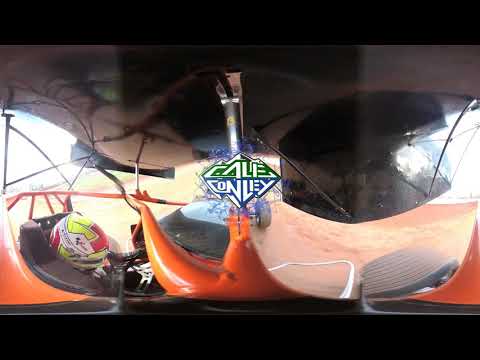The image depicts Cale Conley, a stock car driver, seated in an orange sand buggy-like vehicle, possibly a specialized drag racer. He is wearing a multicolored racing helmet and is viewed from above, giving a top-down perspective inside the vehicle. The background reveals a sandy or desert terrain. In the center, there's a prominent logo displaying the name "Cale Conley" in white font with green and blue outlines. A large, roof-like structure can be seen overhead, casting shadows, and what appears to be a large, borderless screen is visible in the upper right portion of the image. The overall scene suggests a high-energy racing environment.